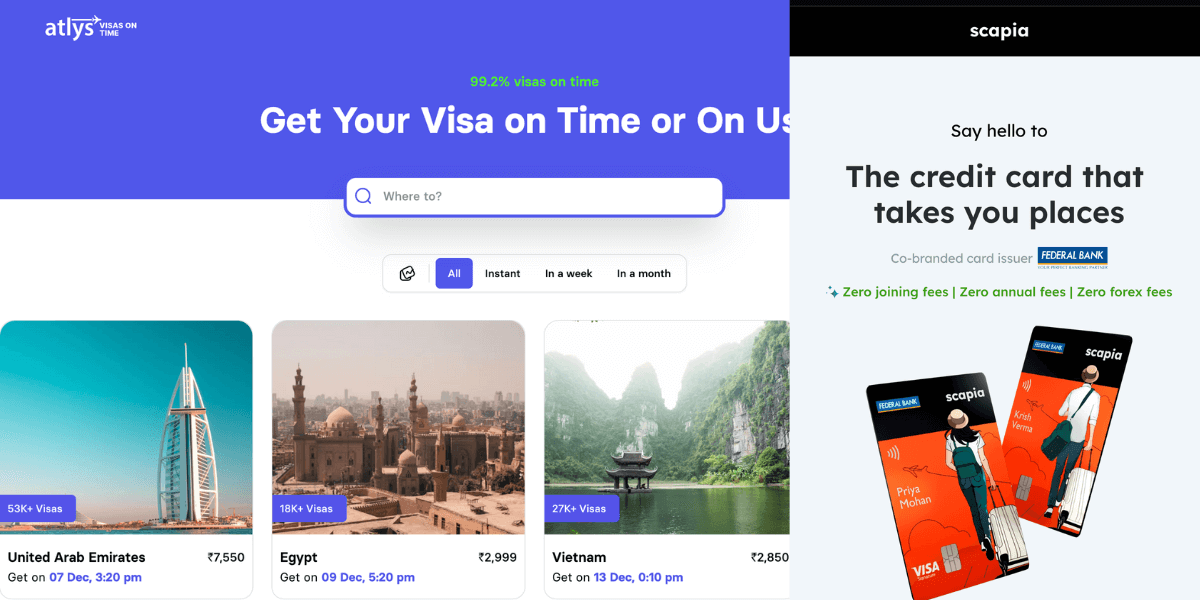The image appears to be a screenshot from a website that is divided into two sections. On the left side of the screen, there's a purple banner with the text "ATLYS" in white print, followed by the tagline "Visas on time." It also highlights two statistics: "92% visas on time" in green font and "99.2% visas on time" in white font below. Beneath this, another line in white font says, "Get your visa on time or on us," accompanied by a search bar labeled "Where to."

Below the banner and search bar, three travel destinations are listed with corresponding details:

1. **United Arab Emirates**: Price is listed as 7550, with a departure date of 07.12 at 3:20 PM.
2. **Egypt**: Price is listed as 2999, with a departure date of 09.12 at 5:20 PM.
3. **Vietnam**: Price is listed as 2850, with a departure date of 13.12 at 1:10 PM.

On the right side of the screen, there's a section with a black border at the top that reads "SCAPIA." Within a grey background and black print, the text promotes a credit card with the message, "Say hello to the credit card that takes you places." It lists the attributes of the co-branded card issued by Federal Bank, highlighting "Zero joint fees, zero annual fees, and zero forex fees." This section also features images of two credit cards from the company.